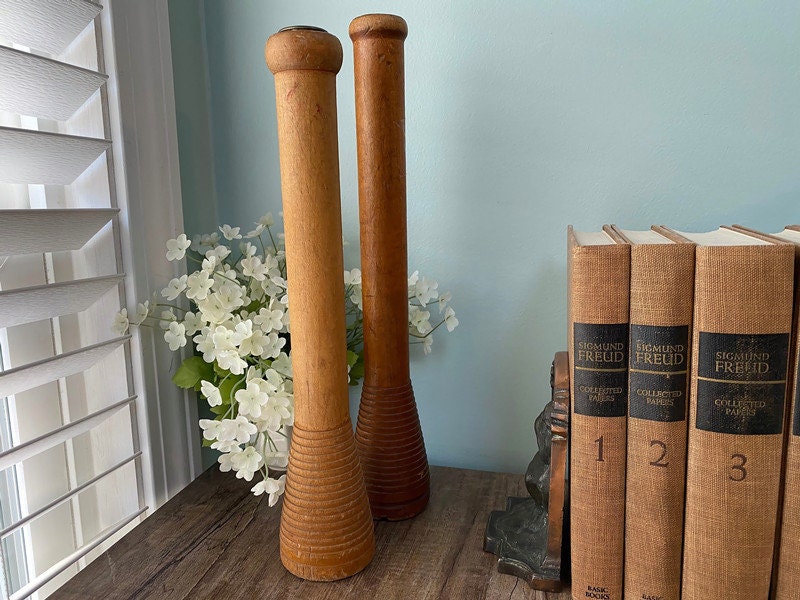The image captures a cozy corner of a home with a light bluish-gray wall meeting a white-trimmed window adorned with plantation shutters. In front of the window sits a rustic wooden shelf made to look like reclaimed barn wood. On the shelf, there is a neat arrangement of Sigmund Freud's collected papers, with three full volumes and part of a fourth, each with a black label on the spine. They are held together by a bronze bookend. Next to the books, there are two tall, decorative wooden spindles, reminiscent of elongated salt and pepper shakers, featuring ringed bases. Adding a touch of nature and contrast, a small vase holding white flowers and green leaves is placed in the far corner of the shelf, completing this thoughtfully designed nook.